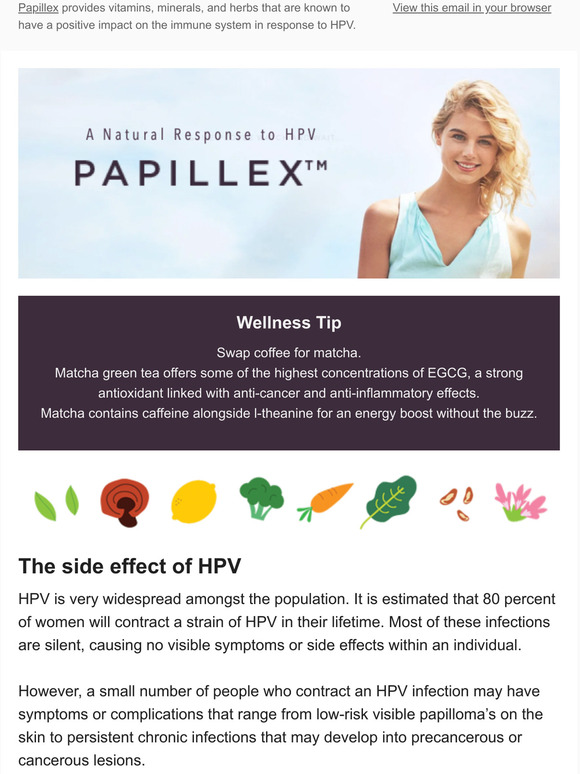This webpage from PAPILEX features a vertical rectangular layout. At the top, a light gray banner spans across the screen, stating in gray text, "PAPILEX provides vitamins, minerals, and herbs that are known to have a positive impact on the immune system in response to HPV." To the right of this text, there's a clickable, underlined phrase, "View this email in your browser."

Below this banner, a horizontal rectangular photograph showcases a slender, blonde woman with long, wavy hair. She is smiling gently at the camera, dressed in a white V-neck sleeveless top. The backdrop is a light blue sky, giving the impression of a sunny day. Overlaying the image, in purple text, are the words, "A natural response to HPV," and underneath that, in dark gray capital letters is "PAPILEX™."

Beneath the photograph, another horizontal box is visually distinguished by its dark purple background. Here, in bold white text, the heading reads, "WELLNESS TIP." Following this heading, additional lines in white text offer a health suggestion: "Swap coffee for matcha. Matcha green tea offers some of the highest concentrations of EGCG, a strong antioxidant linked with anti-cancer and anti-inflammatory effects. Matcha contains caffeine alongside L-theanine for an energy boost without the buzz."